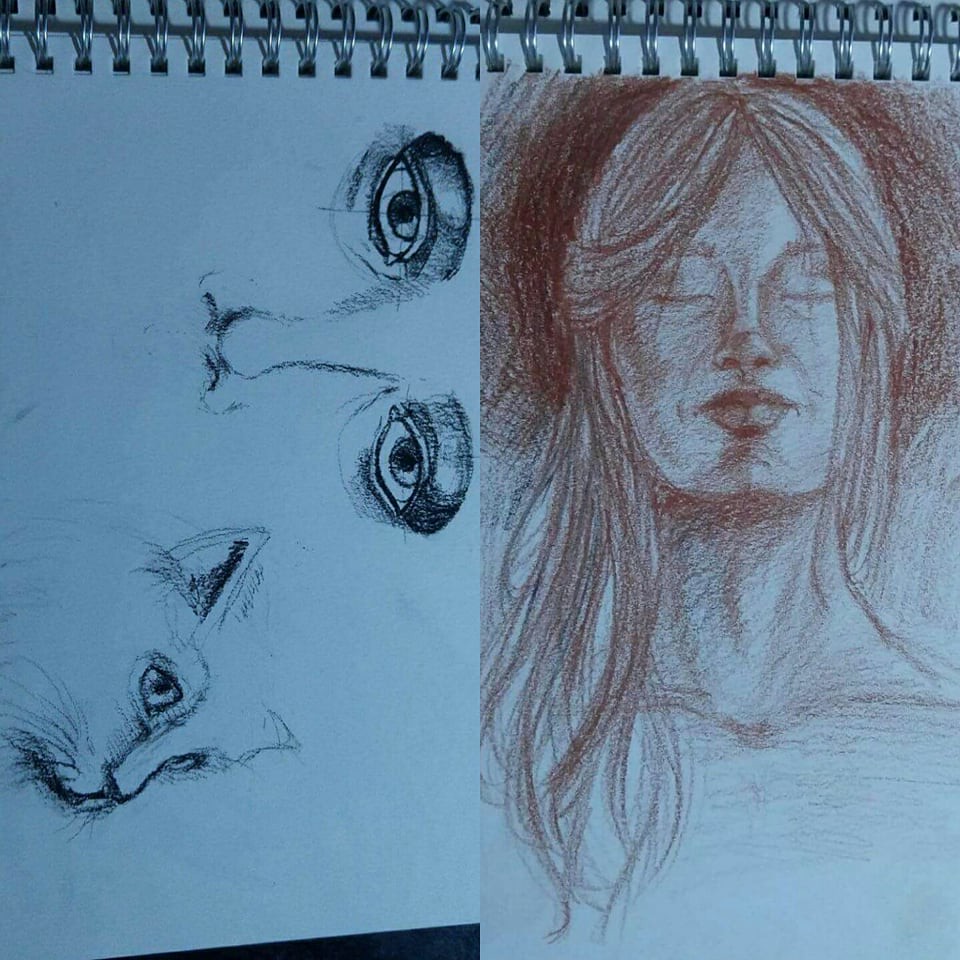The image features two distinct sketches placed side by side, likely created with pencil or charcoal. The left sketch, oriented vertically, showcases a close-up of a human face in black and white, focusing on the bold eyelids, nose, and part of the lips. Below the face, there is a detailed sketch of a cat's head with pointy ears, nose, eyes, and whiskers. The right sketch, rendered in brown and red hues, depicts a woman's full face and neck, with long hair cascading past her shoulders. Her eyes are closed, and she possesses an upturned nose and full lips, with significant shading and details around her neck, face, and hair. The sketches are presented on sketch pads, complete with visible holes and metal rings at the top right, adding to the tactile realism of the scene.